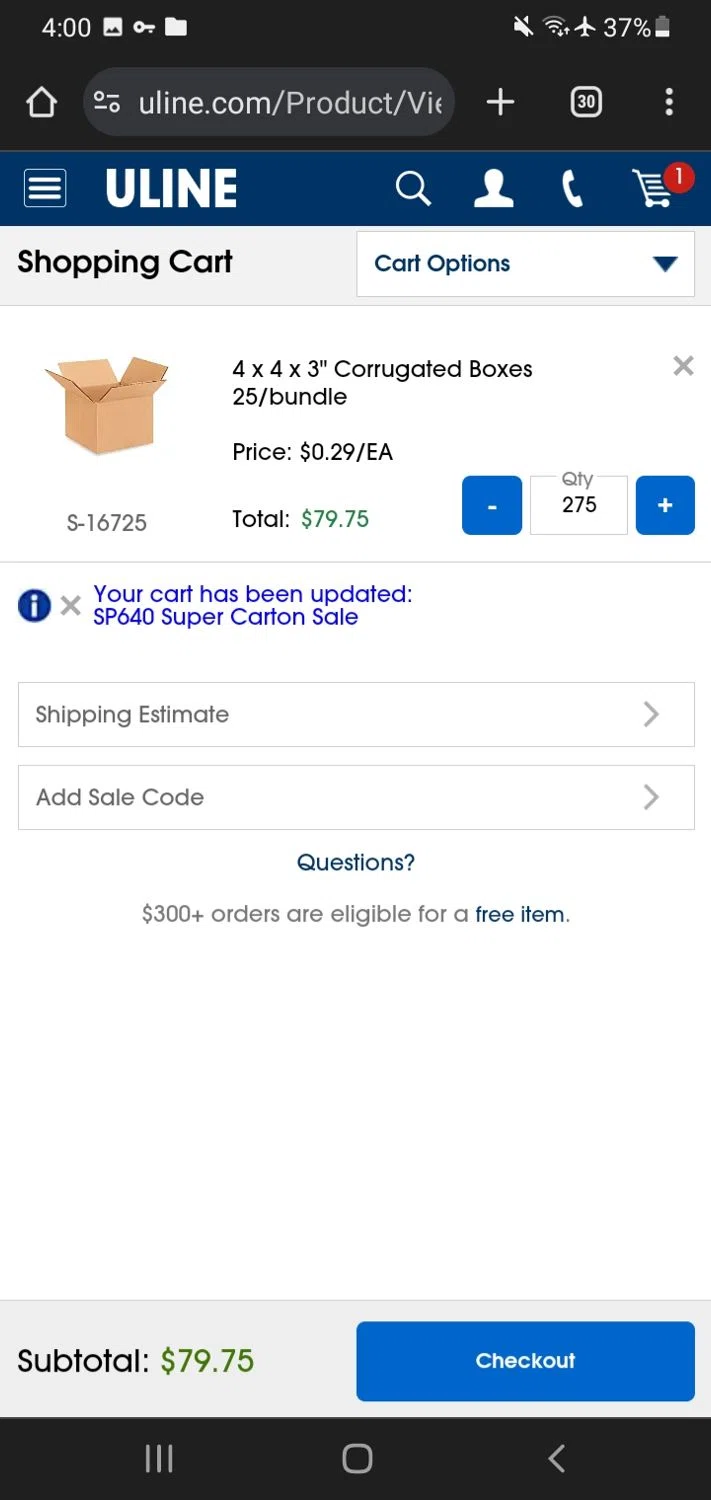The image depicts a detailed screenshot of an online shopping cart on the ULINE website. The top of the page shows the system time as 4 o'clock, with icons for a key, folder, speaker, and wifi signal, all fully connected, indicating a strong internet connection. The airplane mode icon is visible alongside a battery indicator displaying 37% charge.

The main part of the image is focused on a specific product: a cardboard box with the dimensions 4 by 4 by 3 inches. The boxes are described as "crooked" and sold in bundles of 25, each bundle priced at $0.29. The total price for the order is $79.75. The interface includes various standard e-commerce controls such as a magnifying glass for search, a person's profile, a phone, a headset indicating customer support, and a shopping cart icon. There are options to update the quantity and the cart itself, which currently reflects a quantity of 275.

The image also includes a command stating "ULINE" at the top and a specific reference code "sb640" indicating the product code or a shipping estimate. There are prompts for entering a discount or promo code, and a note that orders over $300 are eligible for a free item. The subtotal is confirmed as $79.75, leading to the final checkout option.

At the bottom of the image, a black bar spans across with faint indications of icons or a design pattern, labeled as "line, line, line, square, and left." The background of the webpage is designed to be white, maintaining a clean and straightforward interface commonly associated with ULINE’s construction supplies and shopping experience.